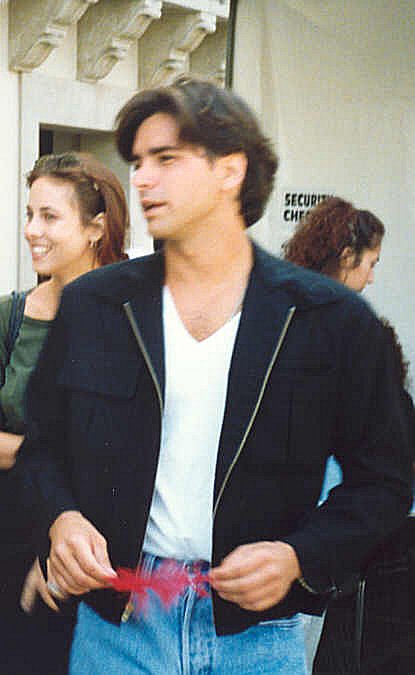In the image, a young man resembling John Stamos is positioned directly in the center. He has medium-length, thick black wavy hair with bangs framing his face, dark eyebrows, and his head is turned slightly to his right, creating a blur effect due to the movement. He is dressed in a white v-neck t-shirt, a black jacket, and light-colored blue jeans, and he is holding a feather or possibly something red in his hands. 

In the background, on the left side, there are two women. One, with brown hair and wearing a grayish olive shirt, is smiling and looking in the same direction as the man, presumably to the left of the image. Behind her, another woman with curly brown hair pulled back is positioned slightly above the man's right shoulder and is looking downward. 

The setting appears to be outdoors in broad daylight, which suggests the possibility of it being on a movie or TV show set. The backdrop features a white or cream-colored facade of a building with architecturally unique ledges or stones protruding slightly. A partially visible sign with the letters "S-E-C-U-R" followed by the beginnings of "I-T" and below that "C-H-E" can also be seen on the wall. The scene is devoid of any other text, and the predominant colors in the image include black, white, red, blue, green, and tan.